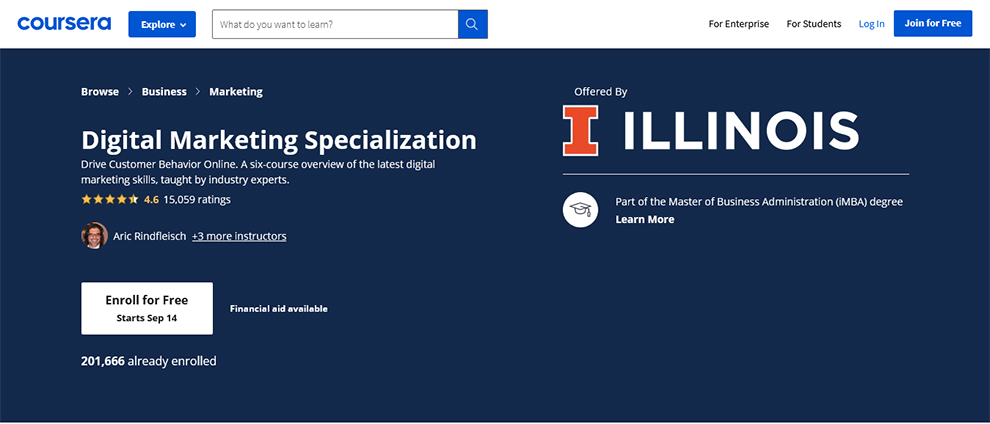This is a detailed screenshot of the Coursera website. The top title bar of the website features a white background, with the Coursera logo prominently displayed in blue letters. To the right of the logo, there is a blue "Explore" button with a drop-down menu. Following this, there's a search box accompanied by a blue button with a search icon. In the upper right corner of the page, there are several navigational links: "For Enterprise," "For Students," a "Login" button, and a blue "Join for Free" button.

In the main section of the webpage, the course is marked as “Offered by Illinois,” with a large, red-filled letter "I" representing Illinois. The left side of the page showcases the title “Digital Marketing Specialization” and states that the course is instructed by Eric Roddenfish. Directly below this, a prominent white button reads "Enroll for Free - Starts September 14th," and to its right, there is a note indicating "Financial Aid Available."

At the bottom left of the page, a statistic notes that "2,001,666 Already Enrolled," highlighting the course's popularity.